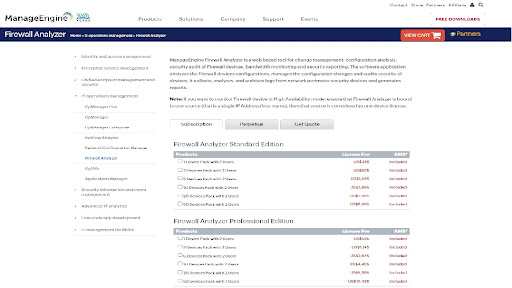The image displays the Manage Engine website interface, with several key sections recognizable despite the poor resolution. In the upper left corner is the "Manage Engine" logo. The top navigation bar contains multiple categories: "Products," "Solutions," "Company," "Support," and an unclear fifth option. On the upper right corner, the menu offers options such as "Free Downloads," a search icon, a profile icon, and a "Create" button, though its exact label is also unreadable due to low resolution.

Below this navigation bar, a blue strip spans the width of the page. On the left side of this strip, “Firewall Analyzer” is prominently displayed in white text. There is additional white text on this strip that is indistinguishable. Towards the right side of the blue strip, there are options to "View Order" and a shopping cart icon highlighted on a red-orange button. Adjacent to this is a yellow label with unclear text.

On the left side of the main content area, there's a vertically aligned navigation column, slightly indented and difficult to decipher. This column contains 16 items listed from top to bottom, but the specifics of each entry are not legible.

Overall, while the structure and color coding of the website elements are partially visible, the poor resolution hampers the readability of finer details and exact text content.